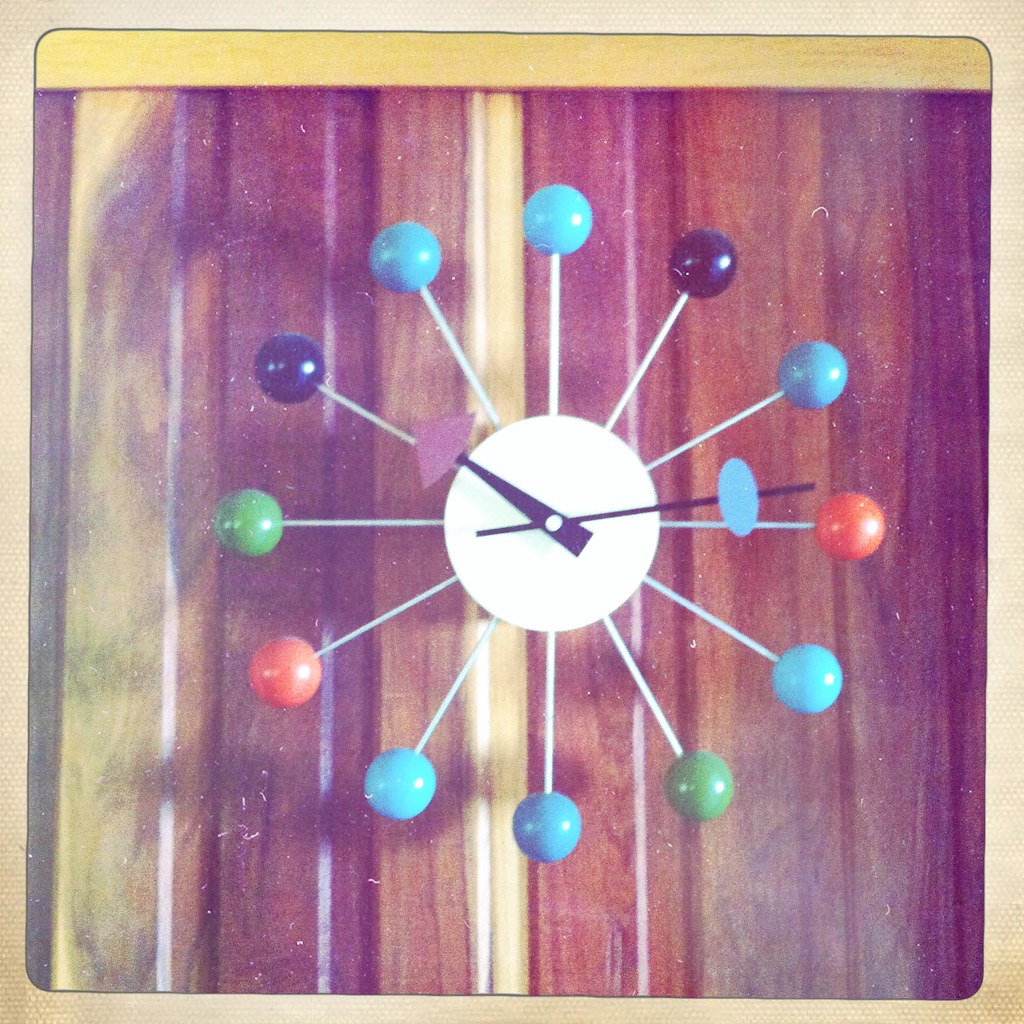The image features a uniquely designed clock without traditional numbers. Instead, vibrant lollipops in various colors - blue, purple, green, and orange - are positioned where the numerals typically would be. At the center of the clock, a white circle holds the black minute and hour hands, with each colorful lollipop radiating outward. The clock is mounted on a wood-paneled wall, showcasing a rich wood grain with an array of brown shades, ranging from light tan to deep, dark hues, adding warmth and texture to the setting.